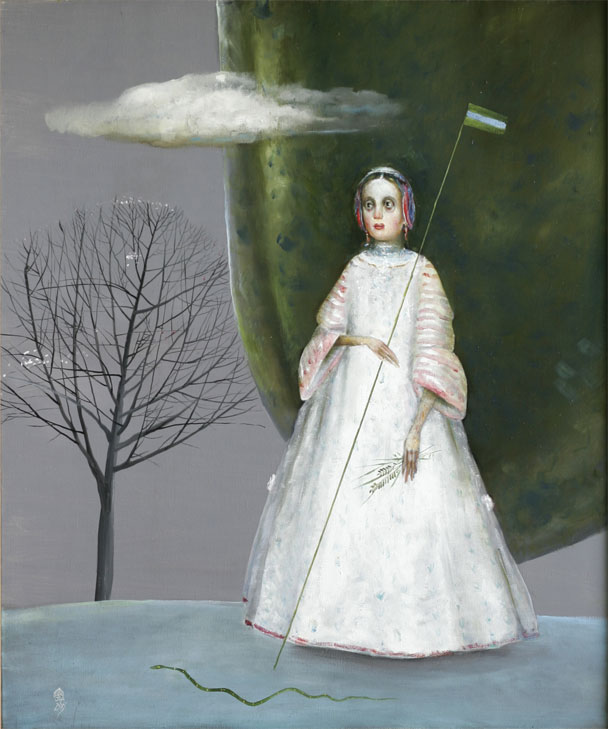This painting is a tall vertical rectangle featuring a wintery scene. On the left side, there is a bare tree with many branches, devoid of leaves, signifying a cold season. The tree stands against a gray background that extends from the middle to the left edge and bottom. Above the tree, a small lenticular cloud floats, its white form outlined in gray. The ground is covered in a layer of snow, illustrated with a white line stretching from left to right across the bottom of the image. Near the center at the bottom, a thin green squiggly shape resembling a snake is visible.

Dominating the right side of the painting is a young woman standing gracefully. She is dressed in a long, flowing white dress with ruffled sleeves tinged with pink, resembling a bell shape that spreads out from her waist. Her brown hair is parted in the middle and covered with a red, blue, and white scarf. She holds a thin pole in her right hand, adorned with a striped flag—green at the top and bottom with a white center stripe. The pole extends over her left shoulder. The woman’s left hand rests on her leg, possibly holding a glove. She also wears earrings and gazes slightly to the left.

Behind the woman, occupying much of the right side, is a large, greenish oval shape that appears almost fruit-like with its green color and blue dots or spots. This object rises from the ground and extends beyond the top edge of the painting. The cold and tranquil scene is set on a snowy, gray-blue background, emphasizing the desolate, wintry atmosphere.